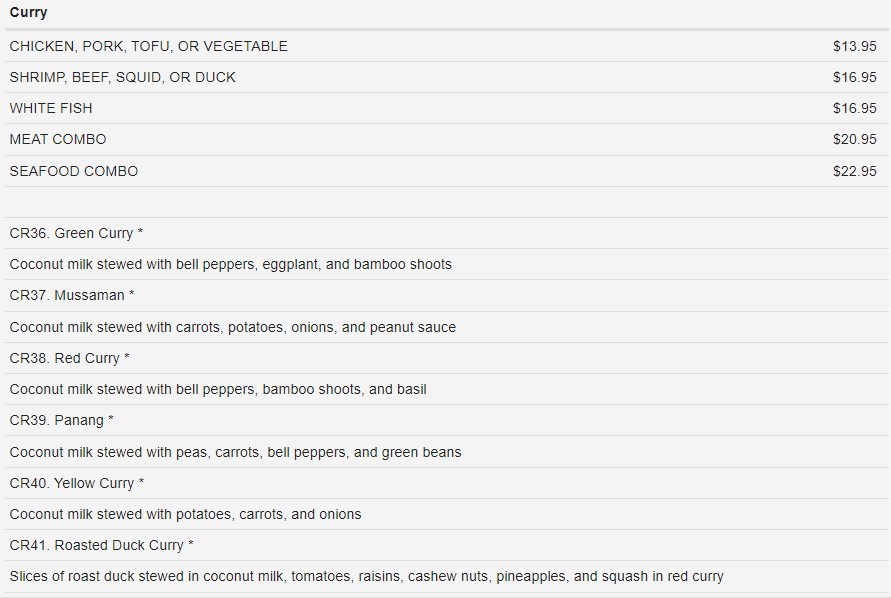**Curry Menu Options**

At the top of the menu, the word "Curry" is prominently displayed in bold letters. Below it, the available curry dishes are listed along with their corresponding prices:

- **Chicken, Pork, Tofu, or Vegetable Curry:** $13.95
- **Shrimp, Beef, Squid, or Duck Curry:** $16.95
- **White Fish Curry:** $16.95
- **Meat Combo Curry:** $20.95
- **Seafood Combo Curry:** $22.95

Beneath the prices, the ingredients for various curry types are described in detail, each identified by a unique code:

- **CR 36 Green Curry:** Contains coconut milk stewed with bell peppers, eggplant, and bamboo shoots.
- **CR 37 Musselman Curry:** Made with coconut milk stewed with carrots, potatoes, onions, and peanut sauce.
- **CR 38 Red Curry:** Includes coconut milk stewed with bell peppers, bamboo shoots, and basil.
- **CR 39 Panang Curry:** Features coconut milk stewed with peas, carrots, bell peppers, and green beans.
- **CR 40 Yellow Curry:** A blend of coconut milk stewed with potatoes, carrots, and onions.
- **CR 41 Roasted Duck Curry:** Contains slices of roasted duck stewed in coconut milk, accompanied by tomatoes, raisins, cashew nuts, pineapples, and squash in red curry.